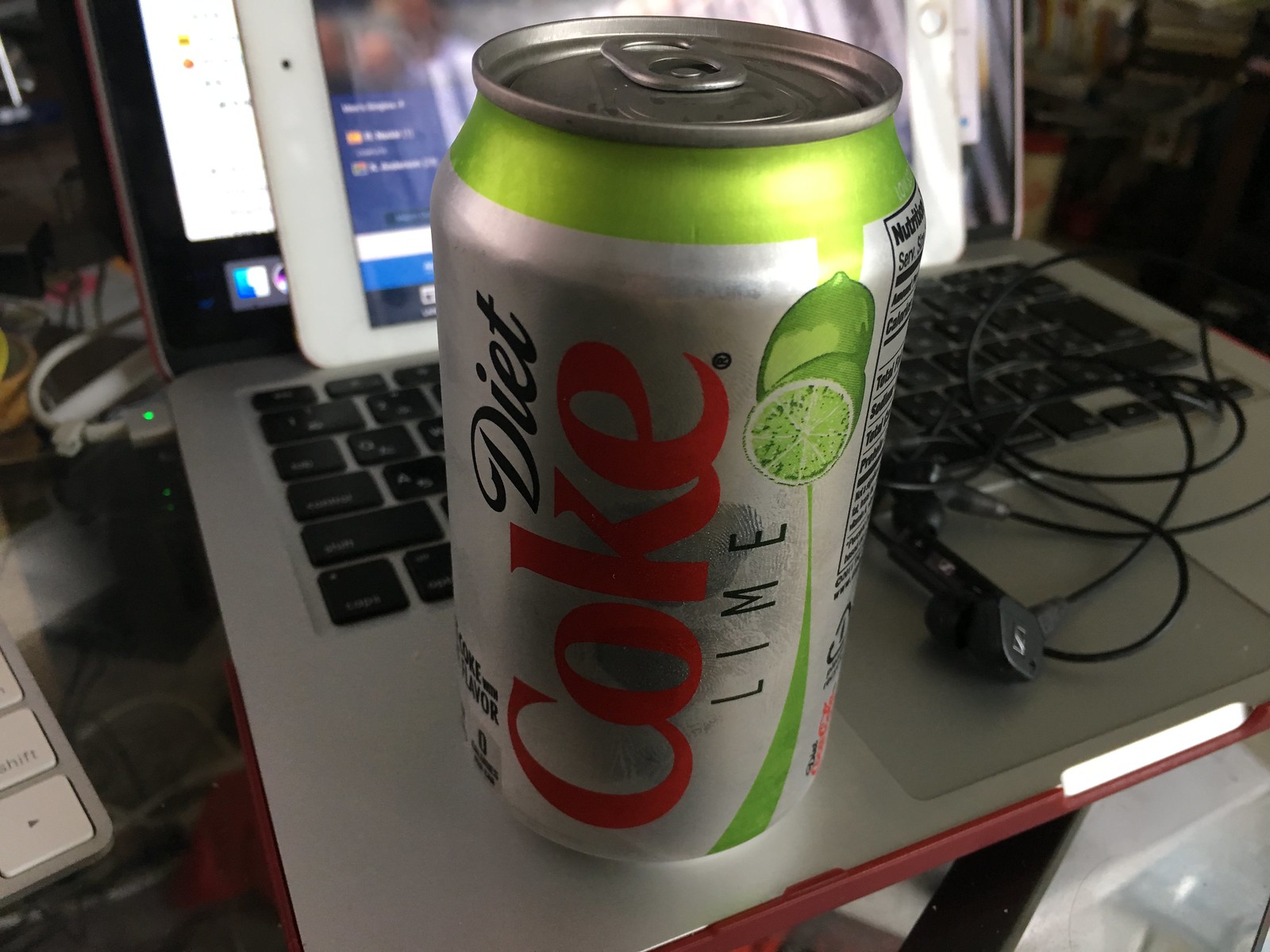The photograph showcases a gray silver laptop with black keys, adorned with wadded-up black earphones laying on the keyboard. A notable feature is an audio jack attachment at the bottom, suggesting the presence of either speakers or a microphone. Leaning against the laptop screen is another screen, likely a tablet or large cell phone, turned sideways. Resting on the base of the laptop, below the keyboard, is an unopened can of Diet Coke in the lime flavor, identifiable by the images of a whole and half lime on its silvery surface. The can's design includes red lettering for "Coke," black lettering for "Diet" and "Lime," and a distinctive lime-colored strip curving around the top. The can appears cold, with visible fingerprints and condensation, raising concerns about potential leakage over the laptop. Surrounding the laptop, the cluttered desk area features glimpses of another keyboard, possibly a number pad or button box, along with various cords and a power strip in the background, illuminated by a green power light.